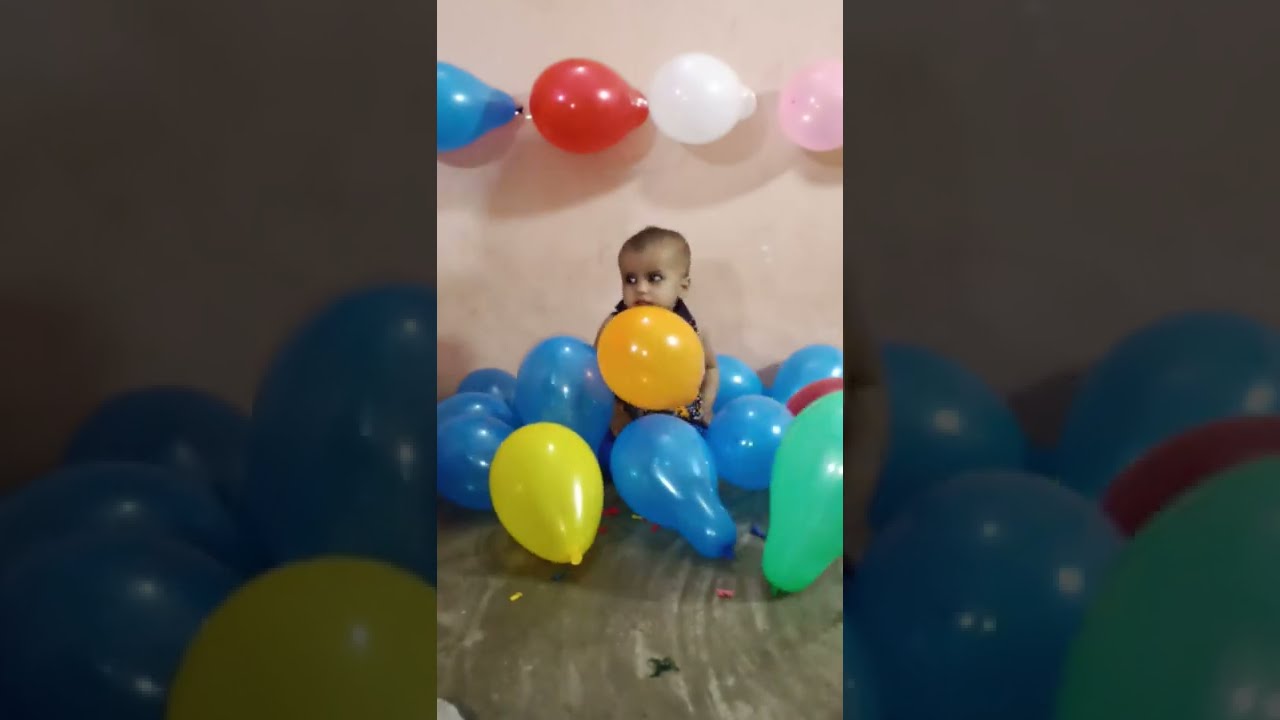In this blurry vertical photo, likely a screenshot from a video, a light-skinned toddler around two years old is sitting on the floor. The floor appears to be gray cement or possibly an olive drab color. In front of a soft pink wall, the child is surrounded by a colorful assortment of balloons. The toddler, who has a neutral expression and is looking off to the left, is holding a large orange balloon that nearly covers his entire body. Scattered around him are mostly blue balloons along with one yellow, one green, and one red balloon. On the wall above, there are blue, red, white, and pink balloons taped in a line. Additionally, the floor is littered with some black, red, and yellow debris, possibly remnants of burst balloons, suggesting a festive atmosphere, perhaps a birthday party.